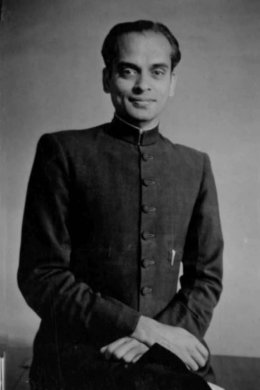This vintage black-and-white portrait showcases a man, possibly from India, seated front and center against a light gray backdrop. He has slicked-back dark hair with a balding top and is clean-shaven. The man exudes a confident demeanor, paired with a sincere, light smile. He is dressed in a button-up shirt or jacket that extends to his neck and has long sleeves. His hands are clasped in a cross-formation over his lap. This photograph, likely from the 1800s, captures only the man in shades of black, white, and gray, devoid of any text or additional objects.